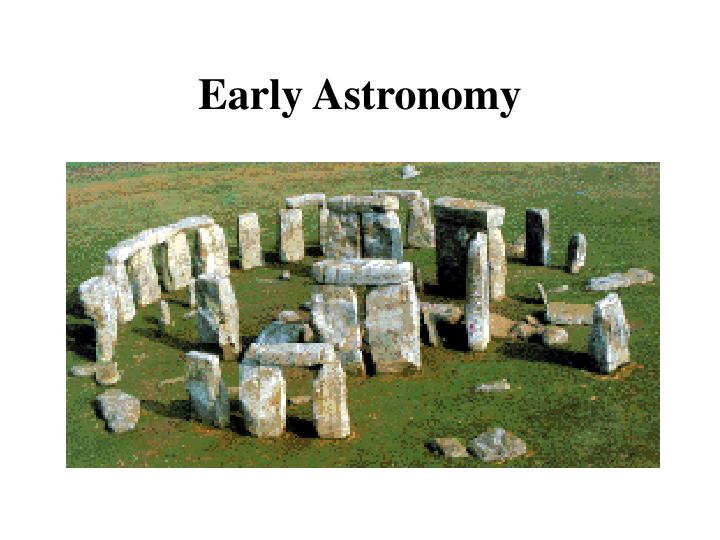The image features a photograph of Stonehenge, set against a white background with the title "Early Astronomy" prominently displayed at the top in black, capitalized letters. The iconic stone arrangement is centered in a flat green field of short grass, captured during daylight. Stonehenge appears as a circular set of monolithic stones, with some stones capped horizontally and others upright or fallen. The stones exhibit hues of gray and brown, adorned with patches of greenish moss. Despite the natural outdoor setting, the overall style of the image leans towards an educational presentation, highlighting Stonehenge’s historical significance in early astronomical practices.